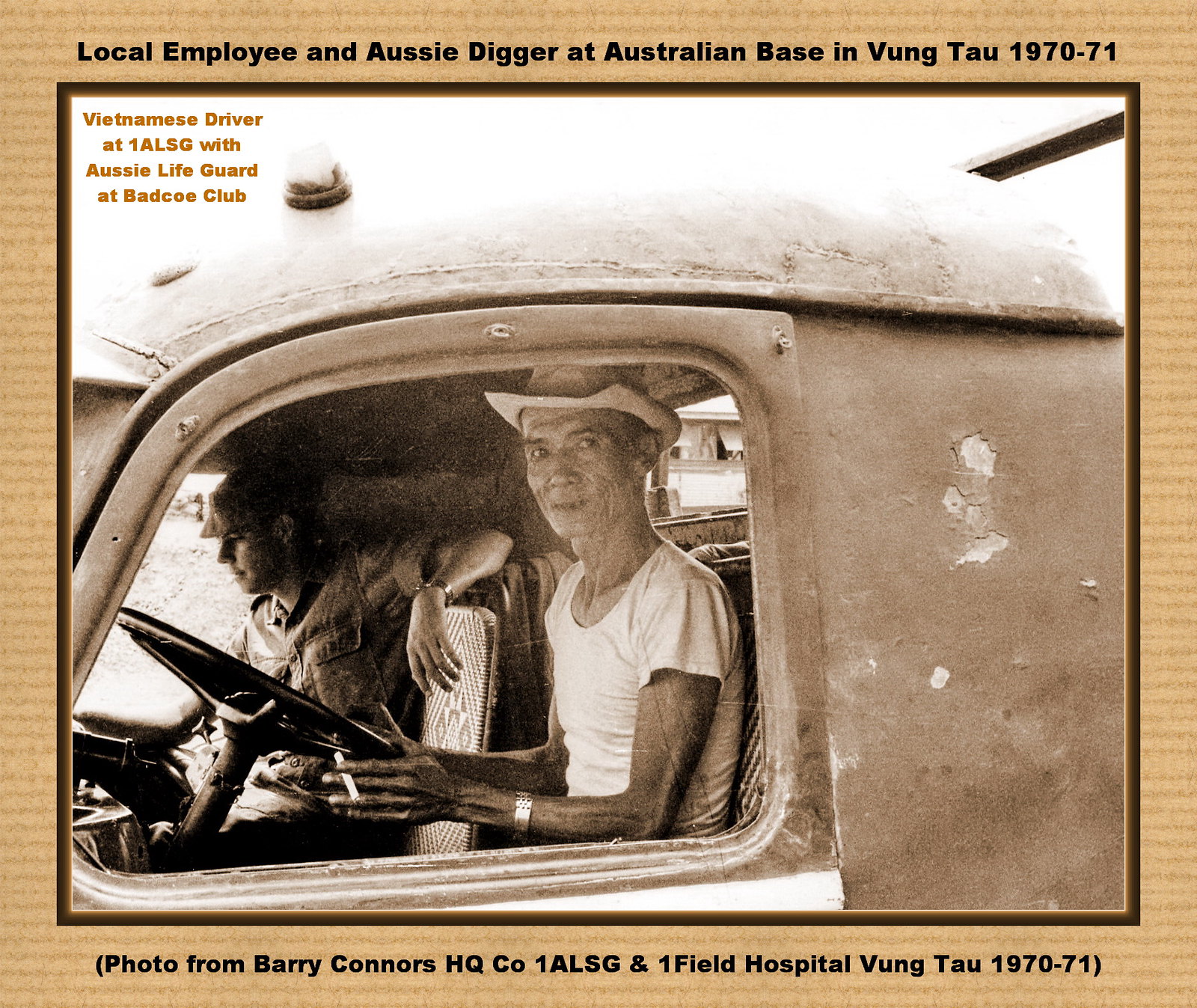This is an old sepia-toned or black-and-white photograph with a tan, beige border. The photograph depicts two men sitting inside a vehicle. The man behind the steering wheel is a thin Asian individual wearing a hat, a white t-shirt, and a metal watch on his left wrist, while holding a cigarette in his left hand. Beside him sits a Caucasian man dressed in a military or official-type uniform, leaning back in the passenger seat and not looking at the camera. The text at the top of the border reads: "Local employee and Aussie digger at Australian base in Vung Tau 1970 to 71." Additional text at the bottom of the border states: "Photo from Barry Connors HQ CO 1ALSG and 1 Field Hospital Vung Tau 1970 to 71." In the top left corner of the photograph itself, the text reads: "Vietnamese driver at 1ALSG with Aussie lifeguard at BADCO Club." This image was likely taken between 1970 and 1971, during the Vietnam War, providing a glimpse into the lives of individuals at the Australian base in Vung Tau.